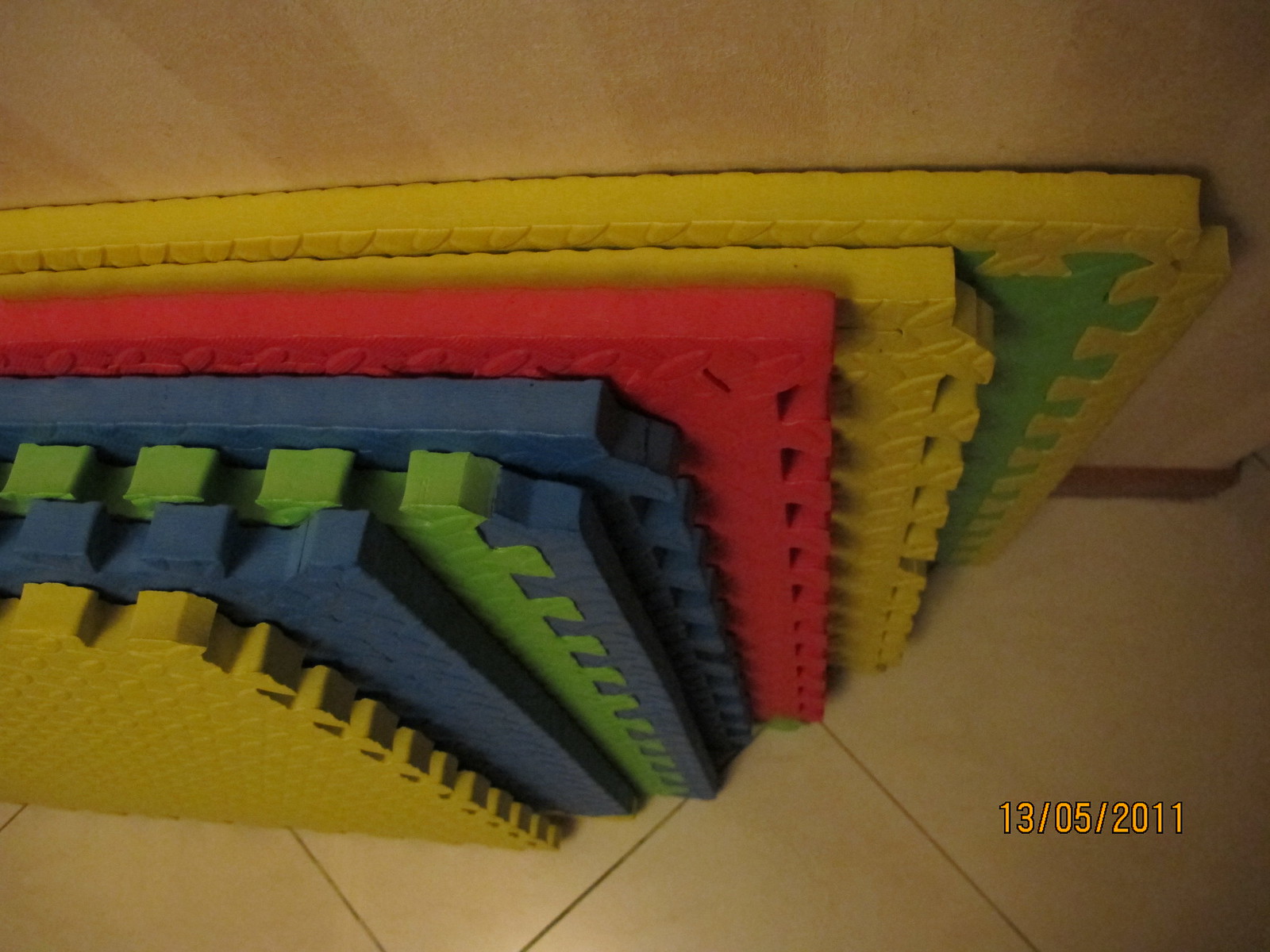The image depicts a set of interlocking foam play mats that are arranged upright, leaning against a faded beige striped wall. In total, there are seven mats of various colors and sizes, including two blue, three yellow, one red, and one green with yellow. These mats are designed to connect like puzzle pieces, creating a soft, safe play surface for children. They rest on a standard beige tile floor. In the bottom right corner, there is a date stamp in orange text that reads "13-05-2011."